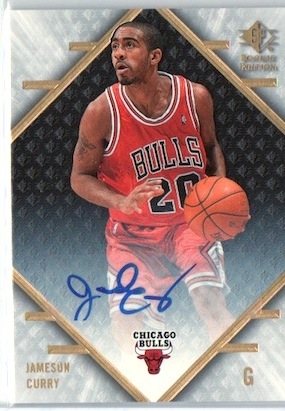The image is a detailed trading card for the Chicago Bulls featuring Jameson Curry, who is prominently centered. Curry, a black man wearing a red Bulls jersey with the number 20, is shown holding a basketball in his left hand, with his gaze directed upwards. The card features a blurry image of him poised as if he is about to shoot the ball. At the bottom left corner, his name "Jameson Curry" is printed in English, and just above this is a "G," indicating his position as guard. In the middle of the card, Jameson's autograph is scribbled in blue cursive, suggesting it was signed by him personally. The card's aesthetics include a gold triangular border around his picture, highlighted by white diamonds. The background is black, with additional colors from his jersey and the basketball's orange. His signature and a Chicago Bulls logo are placed centrally below the image. In the upper right corner, there is a somewhat unreadable logo with a gold embossed design, possibly indicating the card's brand, with some ambiguous text beneath it.